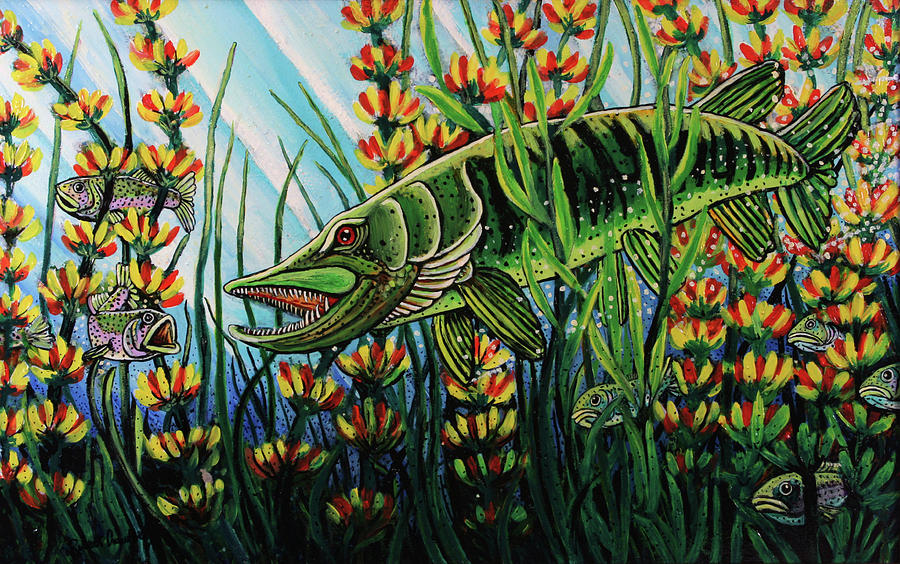This vibrant underwater scene is a painting that showcases a colorful array of marine life. The centerpiece is a large, elongated green fish with striking red eyes and sharp, pointy teeth. Its body features a unique black pattern, and its mouth has a beak-like shape. Surrounding the main fish are smaller fish, green on top and pink on the bottom, swimming randomly through the scene. The underwater environment is filled with lush, long green plants interspersed with flower-like formations that boast yellow and red petals. The background is depicted with shimmering blue water, adorned with white light patterns, bringing a sense of depth and movement to the artwork.